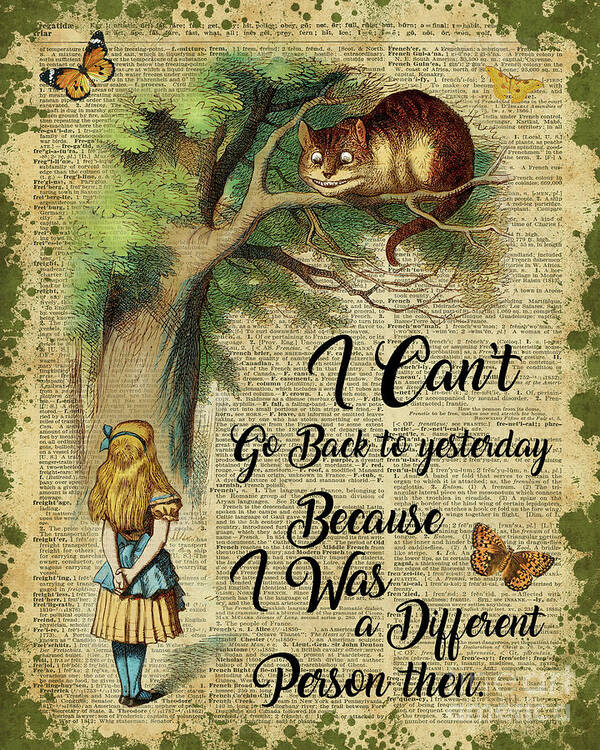The image is a vintage-style illustration based on "Alice in Wonderland," set against a parchment that resembles a page from an old dictionary with the F section of words partially visible beneath. It portrays Alice, identifiable by her long blonde hair, blue dress with yellow accents, and stockings, looking up with her hands crossed behind her back at the Cheshire Cat, who is smiling down at her from a tree. Surrounding them are three monarch butterflies—one in the upper left corner, one in the upper right, and another in the bottom right. Below the tree branches and the cat is the quote: "I can't go back to yesterday because I was a different person then." The borders of the image are spotted green, enhancing the whimsical vintage aesthetic.